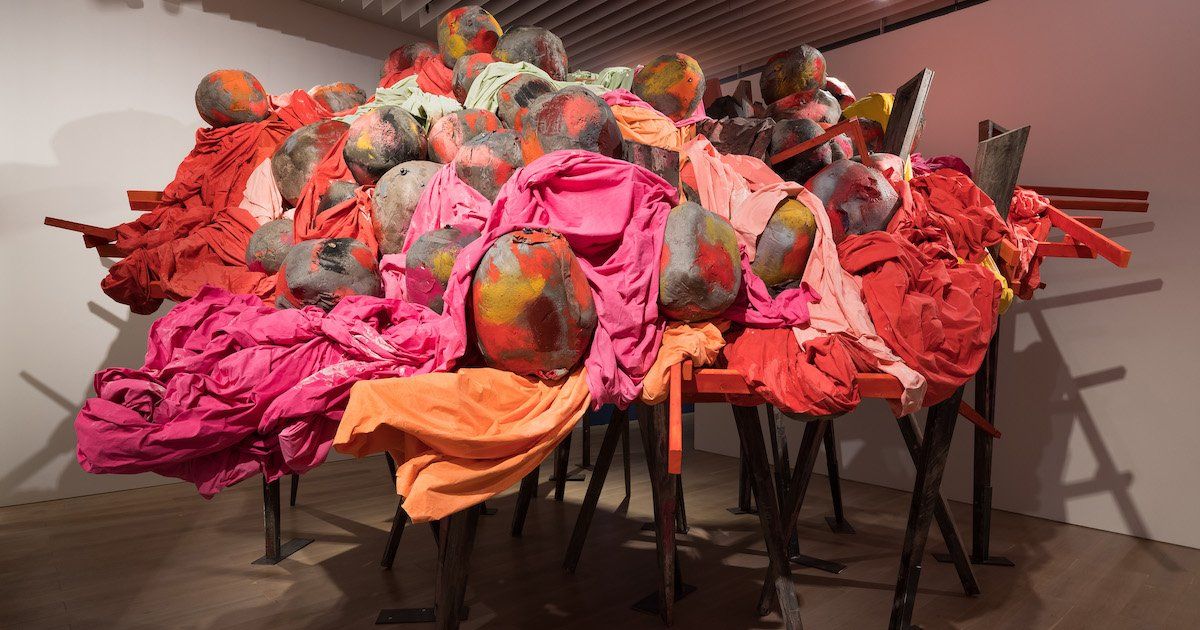This photograph captures an intriguing art exhibit set in the corner of a museum gallery with white walls and brown wooden floors. The centerpiece of this exhibit is an intricate assemblage of roughly spherical objects resembling balls or rocks, possibly even skulls, intermingled with vibrant fabric and paint. These objects, painted with splashes of yellow, red, pink, orange, and cream, are layered and intertwined with sheets of fabric in hues of deep red, light pink, bright orange, hot pink, peach, and minty green. Jumbled together and coiled atop, they evoke an image reminiscent of eggs in a chaotic nest. This entire arrangement is perched several feet above the floor, supported by a complex scaffolding of wooden planks and vertical stilts. This structural lattice features crisscrossing sticks forming Xs, with approximately 20 to 30 legs extending from the bottom, creating an intricate network. The exhibit is illuminated from above, casting varied shadows across the chaotic yet meticulously arranged scene, emphasizing the slotted or lined ceiling above.